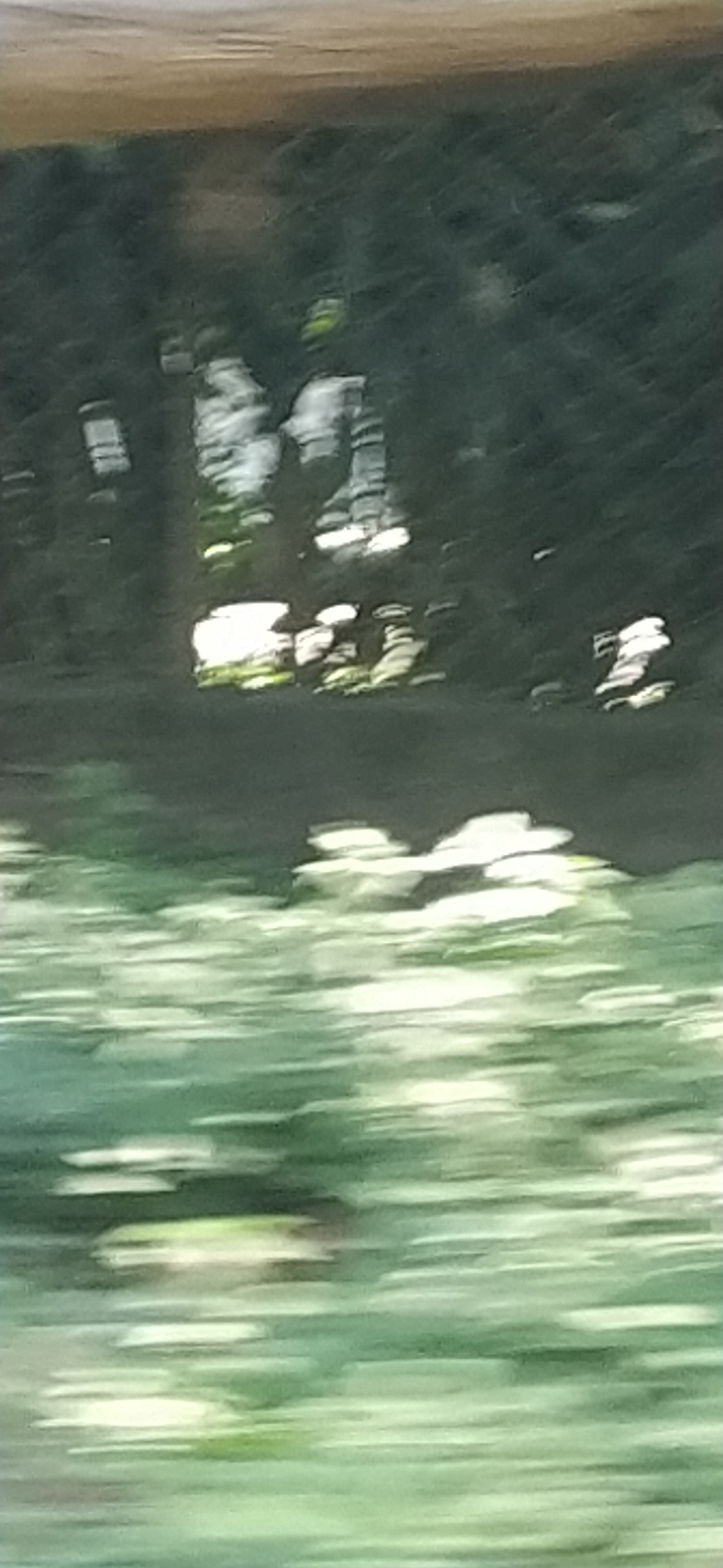The image presents a narrow, tall, and grainy perspective that gives the impression of being taken from a moving vehicle or boat. The bottom half of the picture features a body of water with various shades of green and creamy white reflections, indicating a rough current with small, horizontal waves. Directly above the water, there's a structure that seems to be the underside of a pier, characterized by dark grey and black areas and a light brown wooden beam stretching across the top. Some light filters through this wooden structure. There is also an indistinct presence of a chain link fence, adding to the overall blurred and unclear quality of the image. The photograph's motion blur makes it challenging to pinpoint details with accuracy.